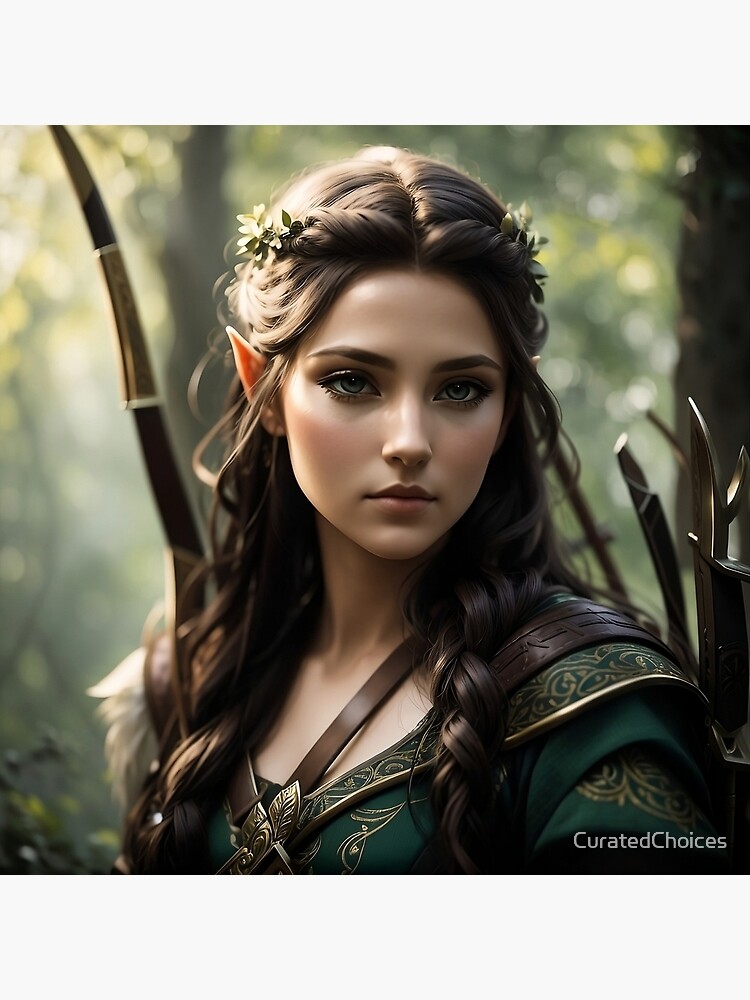The image is a photorealistic computer-generated rendering of an elf-like female with intricate details. She has pointed ears and long brown hair, partially braided into a crown adorned with white and green flowers. Her wide, pointed eyes and thick, pointed upper lip give her an otherworldly appearance. She wears a dark green tunic, intricately embroidered with gold, which extends from her shoulders down to her chest and includes golden accents on her shoulder pads. Two brown leather straps, connected by a golden clasp, crisscross her body.

On her back, she carries a leather satchel containing a quiver of arrows, and she is holding a brown and gold bow. Her eyes are dark, either black or green, and her skin is light. In the background, a blurry, sunlit forest with tall green and brown trees sets the scene. At the bottom right of the image, a watermark reads "curated choices." The overall atmospheric lighting indicates it is daytime in the forest, enhancing the ethereal quality of this digitally-created elf-like figure.